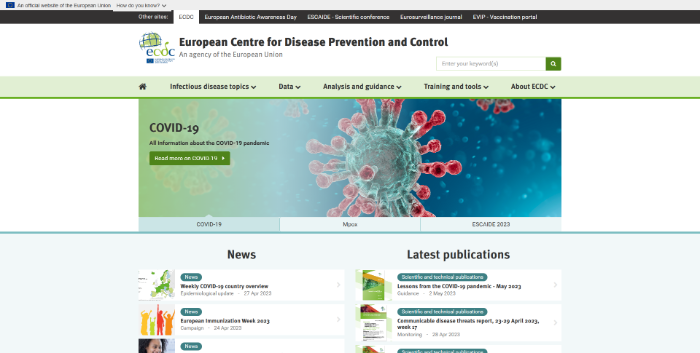A screenshot of the European Centre for Disease Prevention and Control (ECDC) website, showcasing a variety of navigational tabs at the top including links to other sites and the European Antibiotic Awareness Day. The title "European Centre for Disease Prevention and Control" is prominently displayed at the top in black text, complemented by various colors throughout the page, such as green, blue, and red.

To the right of the title, the ECDC logo is visible in blue and green alongside the subtitle, "Agency of the European Union." Below this, several tabs are displayed, including "Infectious Disease Topic," "Data," "Analysis," "Guidance," "Training and Tools," with a search bar situated above them.

In the center below these tabs, the focus shifts to COVID-19, with sections providing comprehensive information about the pandemic. A vivid, detailed image of the virus, primarily blue with red accents, is prominently featured. Underneath the image, text reads "COVID-19 Maps." Adjacent sections include "News" on the bottom left with updates like "Weekly COVID-19 Country," though some text remains indistinct, and "Latest Applications" on the bottom right.

This organized layout reflects the ECDC’s dedication to providing accessible, critical information on infectious diseases, with a particular emphasis on the ongoing COVID-19 pandemic.